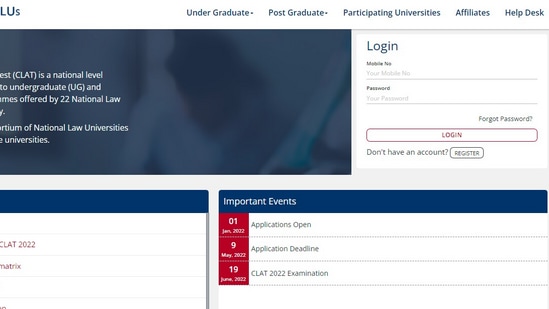This cropped screenshot captures a detailed section of a webpage. 

The header, set against a white background, showcases several navigation options in slightly blue text: "Undergraduate," "Postgraduate," "Participating Universities," "Affiliates," and "Helpdesk," each separated by a dot.

Beneath the header, the main content area has a light grey background. On the left side, there is a very blurry, blue-tinged, and darkened photograph, which is indistinct and cut off by the edge of the frame. Accompanying this image are paragraphs of white text, mostly obscured and unreadable due to the frame's cutoff.

On the right side, overlaid on the light grey backdrop, is a prominently visible white rectangle with slightly rounded corners. At the top left of this rectangle, "Login" is written in blue text. Below this, "Mobile No." appears in small black text, followed by a thin light grey underline and placeholder text in very light grey that reads "Your Mobile No." In a similar format, "Password" is listed beneath, with a light grey underline and the placeholder text "Your Password."

To the right and slightly below these fields, medium grey text asking "Forgot Password?" is right-justified. Below this prompt, a white button with a red outline and rounded corners displays "Login" in red text.

Further down, left-justified medium grey text states "Don't Have an Account?" Adjacent to this text, a white button with a medium grey outline and rounded corners shows "Register" in grey text.

Additionally, there are two sections below this form, each featuring a dark blue header and a white background, though the specifics of these sections are not detailed in the frame.

In summary, the screenshot details a website's login interface with clear textual and structural elements, albeit alongside some obscured and blurry visuals.